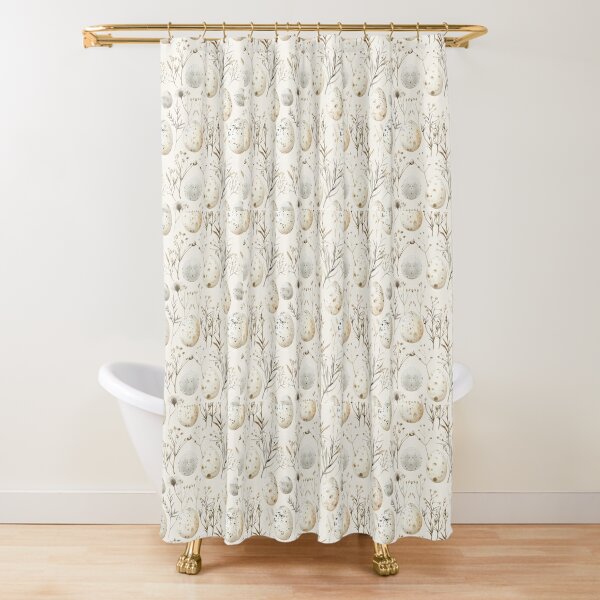This is a photograph of a white clawfoot bathtub with brass or bronze-colored feet, styled to resemble animal claws. The tub is partially concealed by a shower curtain, which hangs from a rod of a similar metallic hue fastened to the wall. The bathtub is situated on a light-colored wooden parquet floor, with white baseboards and a white or slightly off-white background wall. The shower curtain, featuring designs of branches and eggs in light tan and gray tones, is draped in a U or circular pattern, making it the central focus of the image. The curtain rod hardware matches the metallic finish of the tub’s feet, adding a cohesive touch to the overall aesthetic.